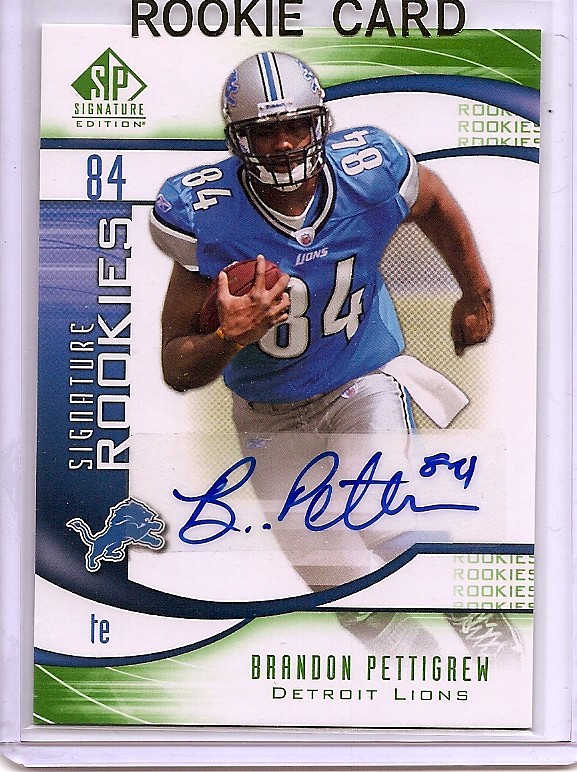The image showcases a rookie football trading card of Brandon Pettigrew, a player for the Detroit Lions. Pettigrew is featured wearing a blue Lions jersey with the number 84 and silver pants, complete with a silver helmet. He is depicted carrying a football in his right arm, suggesting he is in action, possibly running. The card is titled "Rookie Card" at the top in black letters on a white background, and it prominently features a photograph of Pettigrew. To the top left corner, there is a green section with "SP Signature Edition" written in white letters. Below Pettigrew's picture, his name is printed in green, and his autograph appears just above it in blue ink. The Detroit Lions logo is situated to the left of the autograph, and running vertically along the left edge of the card are the words "Signature Rookies 84." The text "TE" indicates Pettigrew's position as a tight end. The card appears to be encased in a plastic protective sleeve, ensuring its preservation. The image's border is white, giving it a clean and striking presentation.